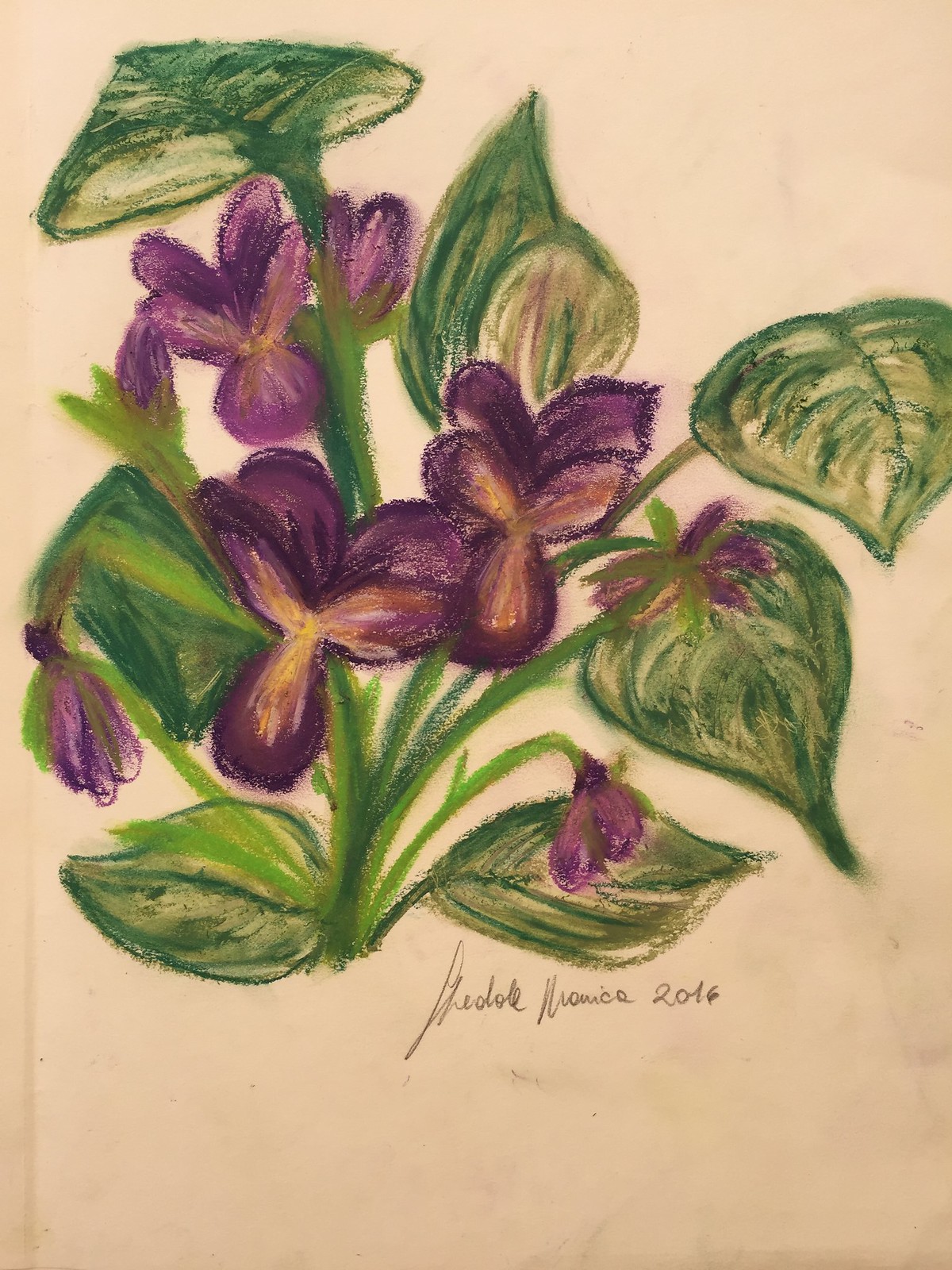A vibrant oil pastel drawing is displayed on a piece of slightly smudged white paper. The smudges, predominantly black as if from charcoal or pencil attempts unsuccessfully erased, frame the main subject - a beautiful purple flowering plant. The plant features large, lustrous leaves that exude a tropical feel. These broad, teardrop-shaped leaves are predominantly green, with touches of white and yellow that add depth and realism. 

Emerging from the lush foliage are dark purple flowers, each with five distinct petals. The petals are adorned with variegated yellow streaks, creating a striking contrast against the rich purple. The composition includes multiple flower buds: three prominent ones and an additional four smaller buds, all contributing to the intricate detail of the drawing. 

Beneath the vibrant florals, the artist’s signature appears in pencil – a stylized cursive script that's somewhat challenging to decipher. It reads "Theolok Moniz" and is dated 2016, providing a finishing touch to this expressive work of art.